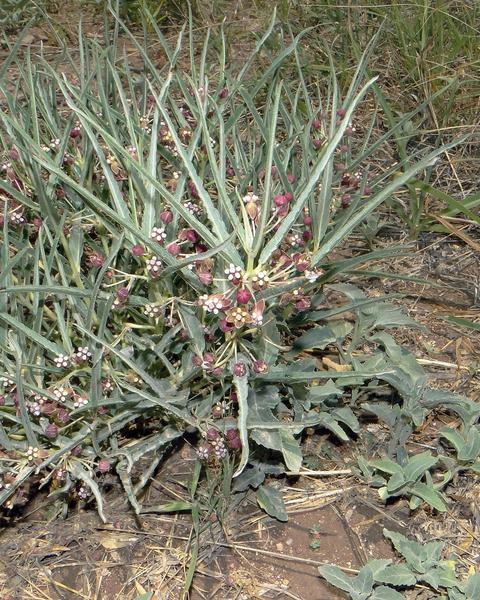This image depicts a vibrant plant emerging from a muddy, brown ground, surrounded by scattered grass and small bushes. The plant is a mix of dark and lighter green hues, with long, pointy leaves reminiscent of a cactus but softer. In the center and extending from the plant are numerous red flowers, each adorned with six small white circles at their centers, indicating they are in various stages of blooming. The plant stands out against a backdrop of dense green foliage, creating a rich contrast between the earthy foreground and the verdant background.